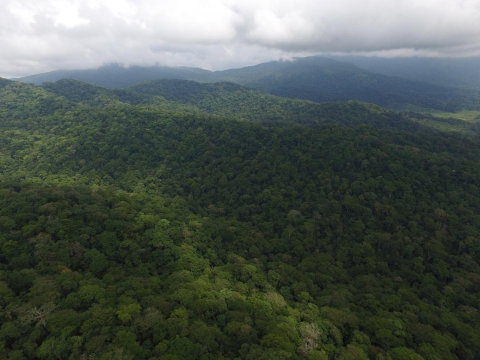The photograph captures a breathtaking landscape of rolling, forested hills taken from an elevated viewpoint, likely from a drone. The foreground is dominated by a vibrant green canopy, showcasing the tops of densely packed trees with varying shades of green, both light and dark. The topography undulates, creating a tapestry of hilly terrain that stretches into the middle ground, where some areas are lit slightly brighter, adding depth to the scene. The distant background reveals steeper, more shadowed hills that fade into a hazy silhouette. Above the hills, the sky is a mix of fluffy white clouds and darker gray ones, with sunlight attempting to pierce through and illuminate patches of the landscape. To the left, lighter clouds catch more of the sun's rays, contrasting with the darker areas to create a dynamic and serene natural setting.